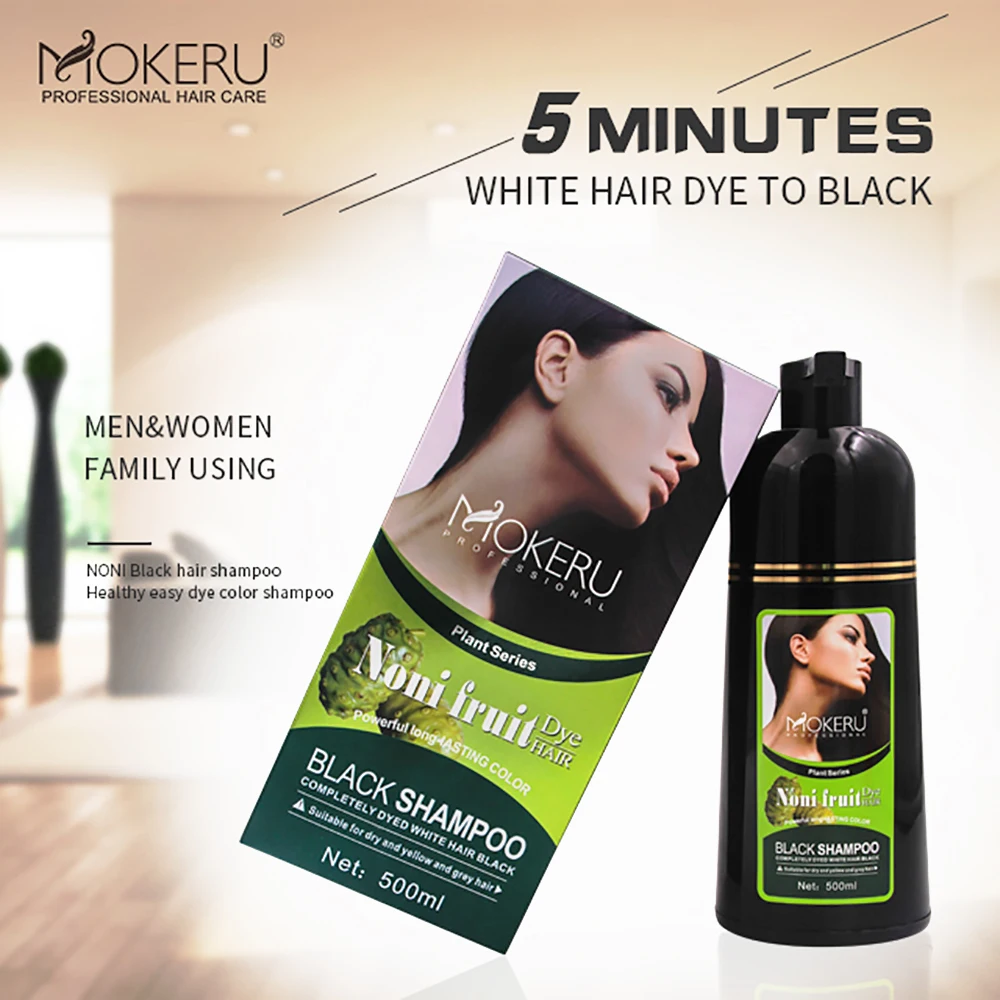This image is a square-shaped advertisement for Moqueru Professional Hair Care's Noni Black Hair Shampoo. The ad prominently features both the product box and bottle, each labeled with "Moqueru Professional Plant Series." The product is a non-traditional, plant-based black hair dye shampoo that promises to transform white hair to black in just five minutes. The packaging highlights its suitability for men and women, and it is marketed as a family-friendly option. Both the box and the bottle display a picture of a woman facing sideways, gazing into the distance. The text on the side of the box reads "Women and Men Family Using Noni Black Hair Shampoo – Healthy Easy Dye Color Shampoo," emphasizing its health benefits and ease of use. The advertisement also notes the product’s powerful, long-lasting color and its suitability for dry, yellow, and gray hair. The net content of the shampoo is 500 milliliters, as indicated on the packaging.